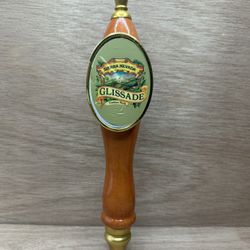The image depicts an ornate beer tap handle, likely seen behind a bar. The handle itself is crafted from shiny medium-colored wood with visible wood grain, and it narrows into a gold-colored metallic end. The design includes a prominent green oval section framed in gold, featuring the word "Glissade" on a gold banner with black text. Above and below the main banner, additional gold banners and a small landscape illustration can be seen. The handle, which curves at various points for ergonomic grip, is set against a textured gray wooden background, adding to the rustic aesthetic. The photograph captures these detailed elements clearly, providing a comprehensive view of the beer tap handle.